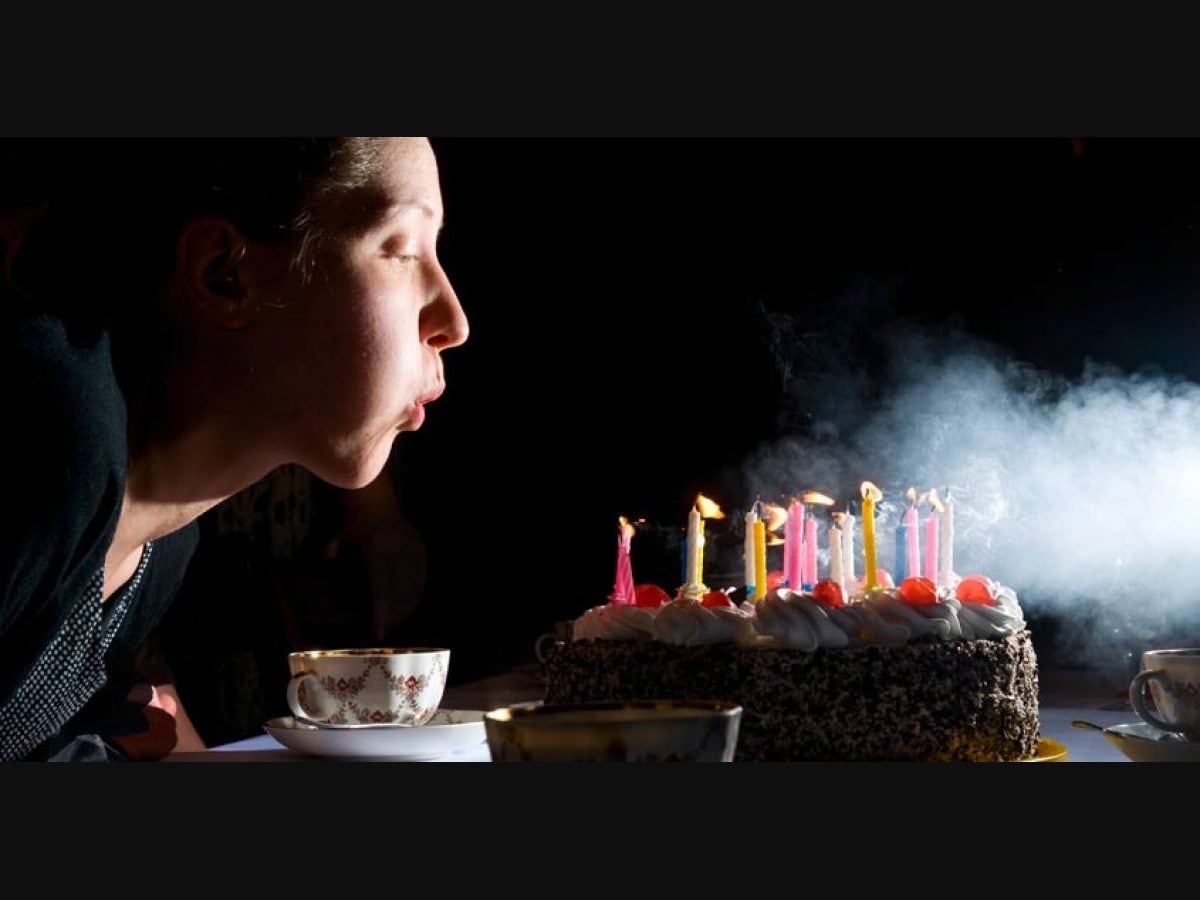The photograph captures a detailed and celebratory scene of a woman, situated on the left side, blowing out an array of multicolored candles on a decadent chocolate birthday cake adorned with swirled white frosting and cherries. The backdrop and parts of the frame are enveloped in black, highlighting the woman wearing a black shirt with a black and white polka dot design. The cake, set prominently on the right, showcases both lit and extinguished candles amidst swirling smoke billowing towards the right. Arrayed around this inviting centerpiece are small teacups, some placed in glass bowls, with one on the far right featuring a spoon on its plate, enhancing the intimate birthday ambiance.